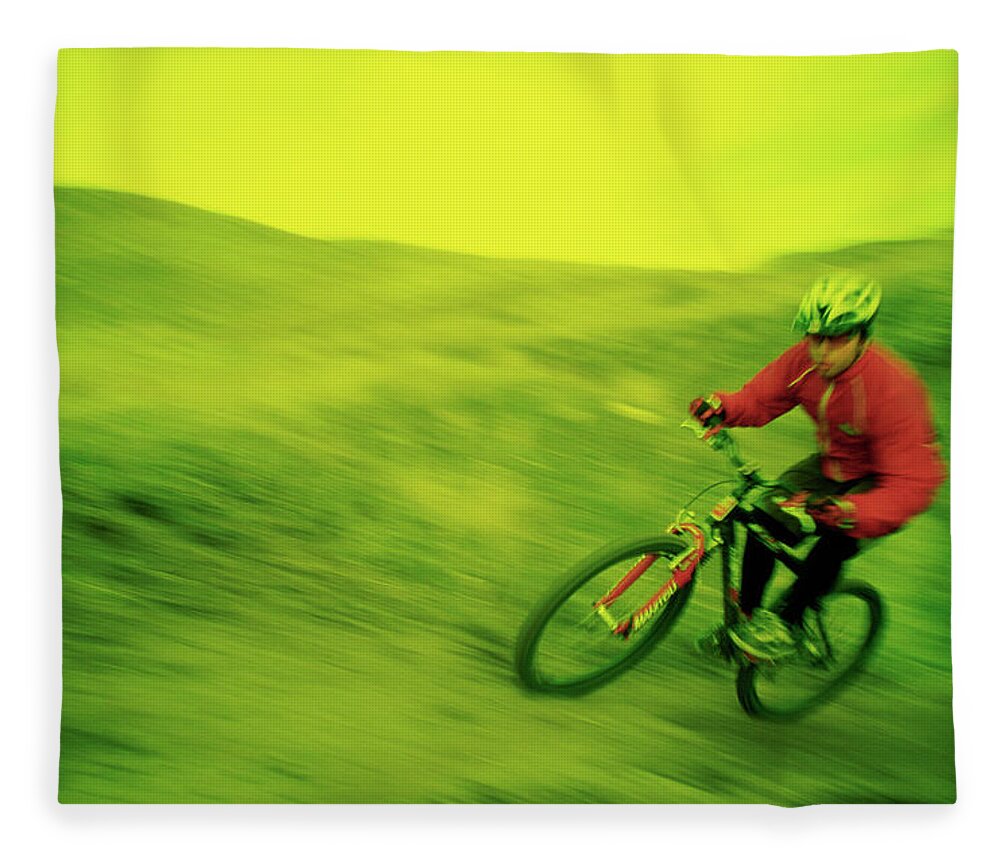The image depicts a dynamic, action shot of a man riding a mountain BMX bicycle, leaning at an angle and seemingly accelerating at high speed. The rider is positioned on a slightly sloped, rugged terrain, which gives the impression of a mountainside or hillside. The entire scene is imbued with a distinctive greenish-yellow tint, as if viewed through a filter, and appears printed on a cloth-like, woven canvas with visible mesh pattern and slight folds.

The cyclist is dressed for the activity with a light-colored helmet featuring black divisions, geometric cycling glasses, and gloves that securely grip the handlebars. He wears a striking red windbreaker with yellow strings at the collar and black pants. His shoes are dark with a white stripe. The bicycle he is riding has a prominent red frame with sponsorship markings, although they are blurred, complementing the action blur effect applied throughout the image.

In the background, the sky is depicted in a gradient of lighter green, contrasting with the darker green of the terrain. This gives the entire image an almost surreal quality, emphasizing the thrill and motion of the high-speed descent on the bike.